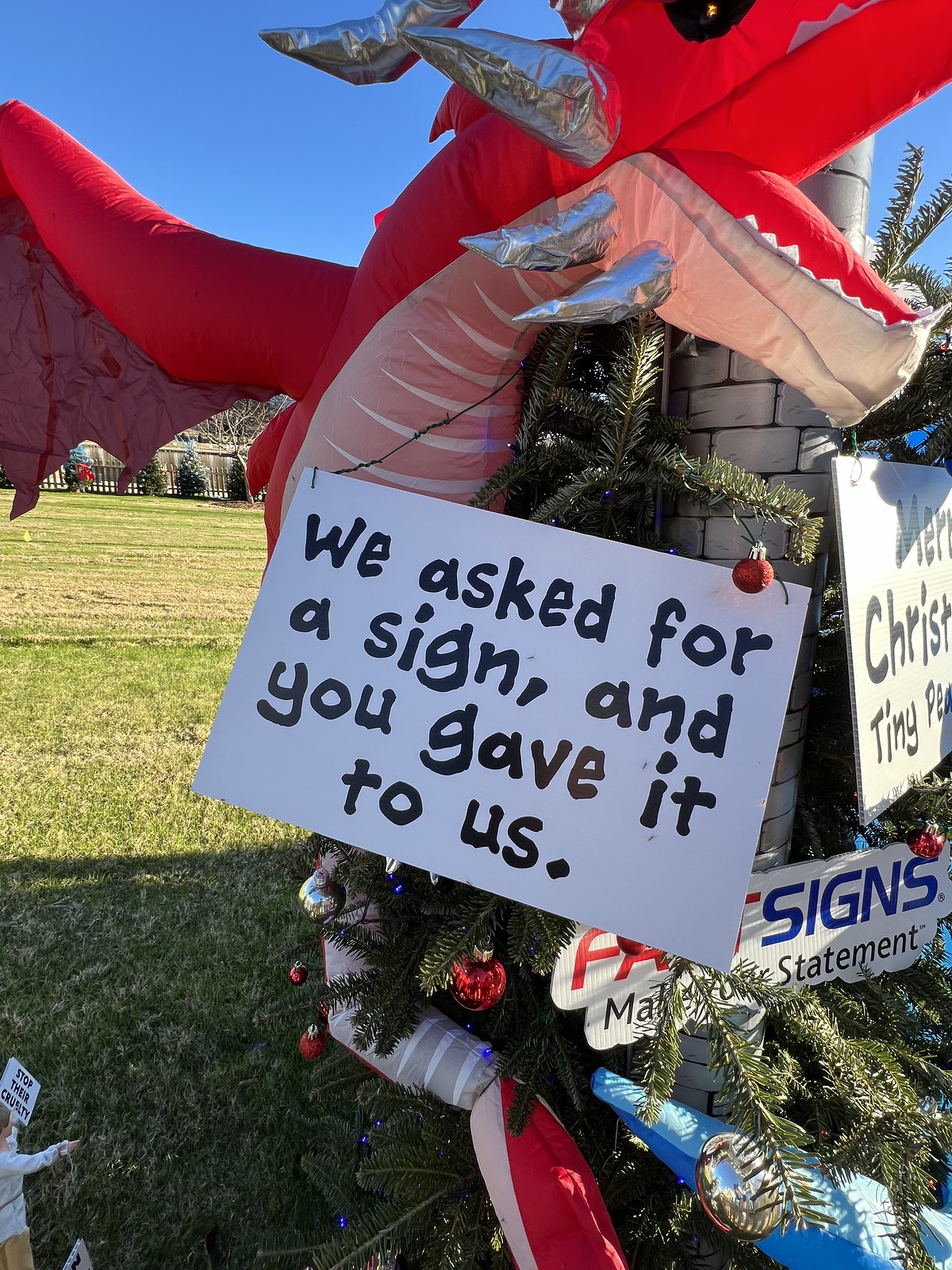In an outdoor setting, standing prominently on a green grassy field under a blue sky, there is a festive display featuring a bright red inflatable dragon with a pink belly, silver horns, and several tusks. The dragon is facing to the right and is wrapped around a structure resembling a brick tower. This structure appears to be placed atop or integrated with a pine tree, which is decorated with an assortment of red, blue, and silver Christmas baubles.

In front of the dragon, there hangs a white placard with black lettering that reads, "We asked for a sign and you gave it to us." Slightly to the right and beneath this placard, there is another partially visible sign, starting with "F.A." in red lettering followed by "signs" in blue. Further right, but harder to see, is another sign that seems to say, "Merry Christmas," with the latter part of the message obscured.

Additional elements in the scene include more pine trees and a fence in the distant background, adding to the outdoorsy atmosphere. In the lower left-hand corner, there is a small doll holding a white sign with the message "Stop Their Cruelty." The entire ensemble conveys a whimsical and festive holiday theme, merging Christmas decorations with a unique and playful centerpiece.